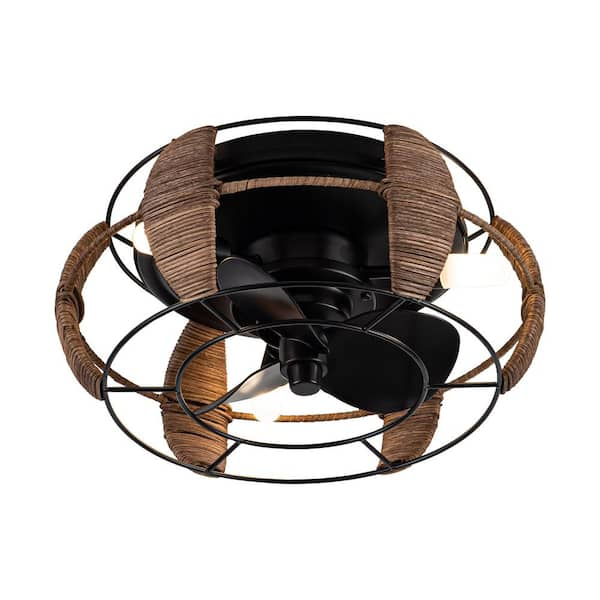The image captures a very unique and modernistic ceiling fan, strikingly set against a plain white background. The fan is designed with a jet-black, circular base, which connects to a larger external frame via several arms. This frame comprises three layers wrapped in a minimalistic wire cage that takes on a hassic shape. The cage is adorned with sections of brown, grainy wood or jute-like rope, adding a decorative and natural accent to the otherwise sleek and industrial design. These earthy materials connect the frame layers, enhancing the fan's aesthetic appeal. Despite its intricate design, the fan is not currently in motion, allowing for a clear, detailed view of its elements. The overall style suggests a custom-made piece, likely requiring a special order, and is characterized by its open-air feel despite the encompassing cage.